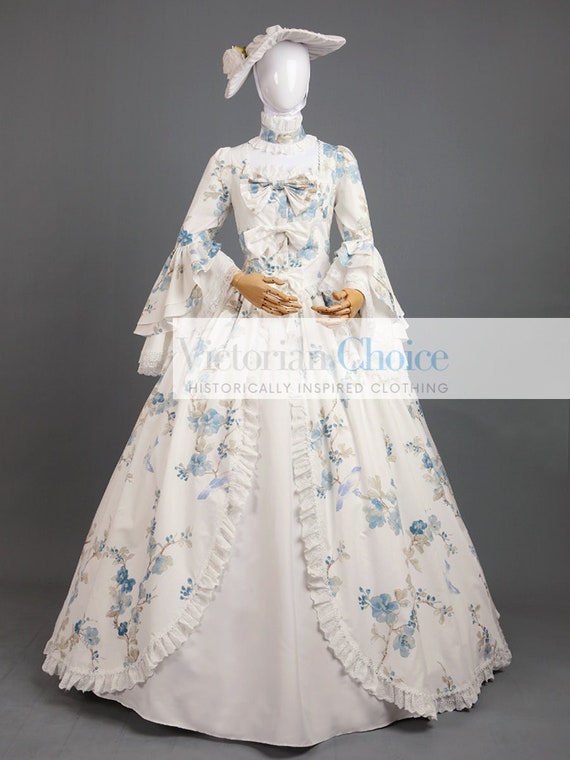The image features a vintage-inspired, ornate white dress adorned with blue and lavender floral patterns, displayed on a full-sized mannequin. The mannequin has a featureless, shiny white head and tan hands with visible joints, positioned near the waist. The intricate dress, reminiscent of the 1800s, boasts long bell sleeves layered with lace peeking out and a full skirt that flares out towards the floor. The front of the dress is detailed with ribbons along the bust. Adding to the ensemble, the mannequin wears a white, frilly, flat hat decorated with flowers, and a matching choker around the neck. An overlay text in a white banner on the right side of the gray background image reads "Victorian Choice Historically Inspired Clothing," with "Choice" highlighted in light blue.